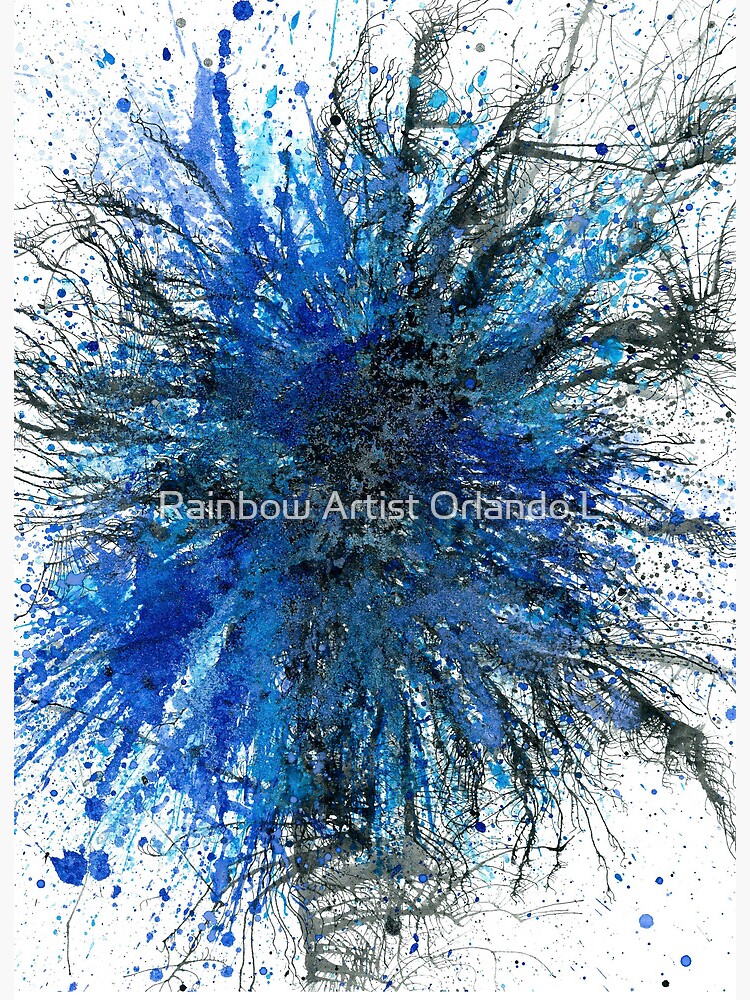In this vibrant painting by Rainbow Artist Orlando, a dynamic blend of various blue shades—bright neon sky blue, cobalt blue, and dark blue—intertwines with bold black splatters on a pristine white background. The rectangular canvas, oriented vertically, features a chaotic yet mesmerizing circular design at its core where the splatters are densest. Radiating outward from the center, the black lines and dots resemble spider webs interspersed with energetic bursts of blue, spreading through hundreds of intricate lines and thousands of tiny specks. A subtle light blue watermark reading "Rainbow Artist Orlando L." graces the middle of the painting, adding a final signature touch to this energetic, Pollock-esque explosion of color and form.